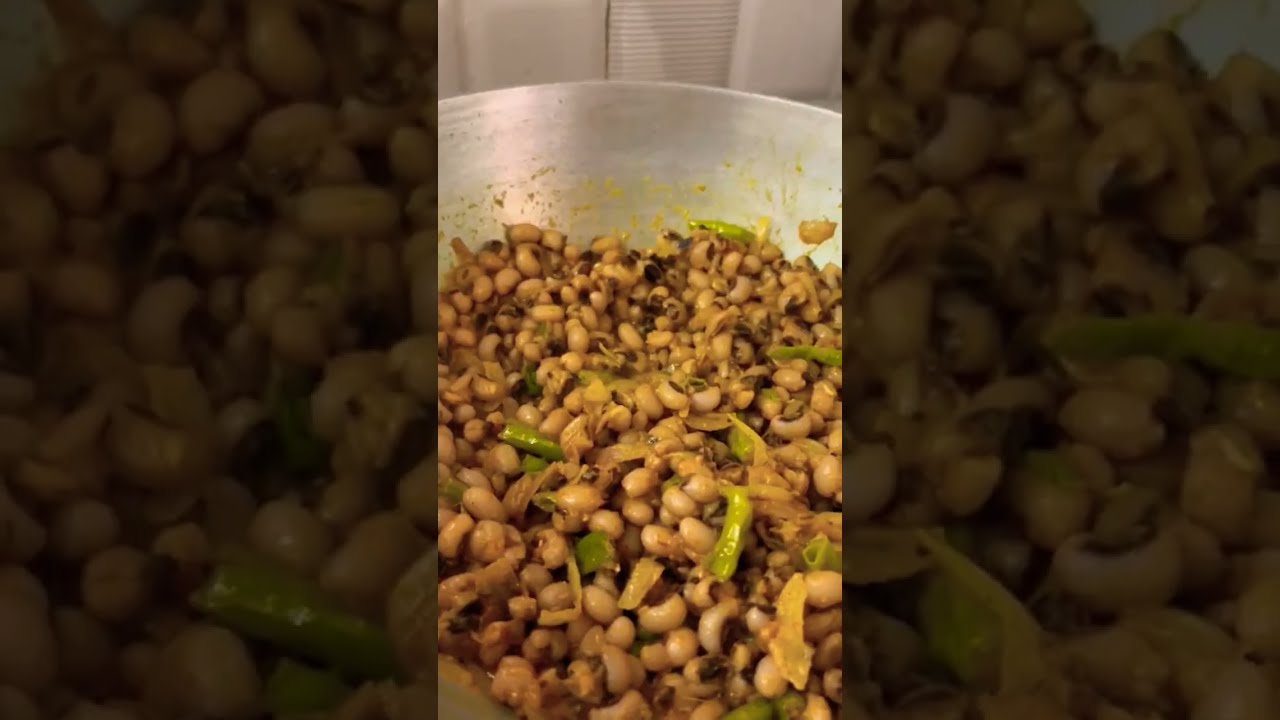This photograph, presented in a vertical, portrait-oriented format, features a vibrant and clearly defined image of a substantial quantity of black-eyed peas, occupying a central position within the frame. These peas are the traditional beige color with characteristic black eyes, and they are nestled inside what appears to be a large stainless steel cooking vessel, likely a wok or a wide pan.

The black-eyed peas are interspersed with chopped vegetables, including discernible pieces of green onion and some form of leafy green, possibly cabbage. The vegetables and peas are densely packed in the center of the vessel. Some of the peas and vegetables cling to the sides, suggesting active mixing or cooking.

The background of the image is blurred, making it hard to discern any specific details, though it hints at a white paneled environment, possibly a kitchen. The foreground image of the peas is significantly sharper and more vivid, creating a strong focus on the food itself. There are no utensils, people, or additional context within the frame, emphasizing the dish's preparation state and the volume indicative of a large recipe.